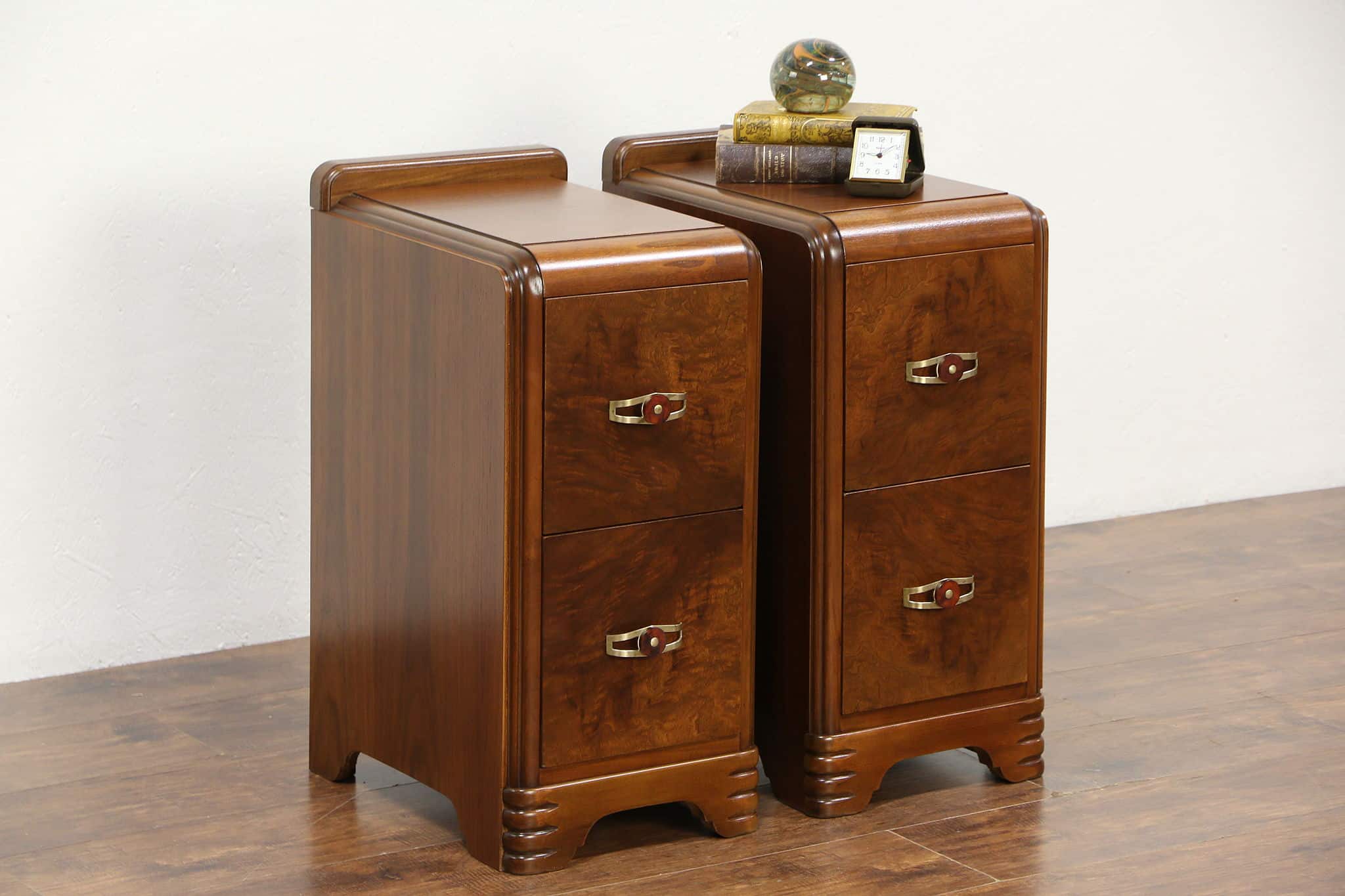The image depicts two identical, high-end miniature cabinets positioned on a hardwood floor against a white wall, evoking a gallery or auction house setting. Each cabinet is rectangular, crafted from polished mahogany wood with a distinct natural grain and adorned with golden circular knobs on the front. The tops of the cabinets are flat with slightly raised edges at the back. The left cabinet stands empty, while the right cabinet holds a neat arrangement on top: two antique books with a crystal ball, resembling a giant marble, placed on top, and a small, vintage travel clock. The refined details and arrangement lend a sophisticated and elegant ambiance to the scene.